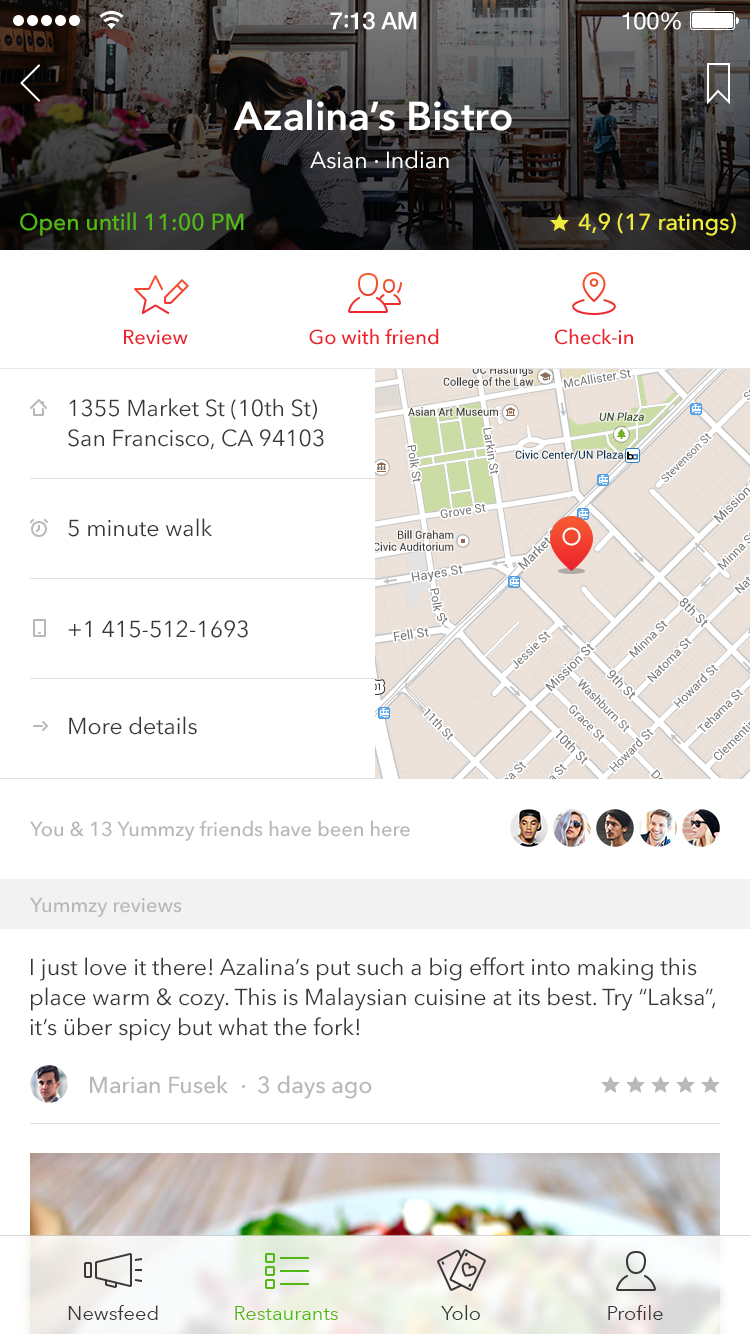This screenshot captures a mobile application's interface focusing on Azzolino's Bistro. At the top of the screen in the status bar, five dots likely indicate full signal strength next to a Wi-Fi icon. The time displayed is 7:13 AM, and the battery indicator shows 100%, all rendered in white.

The background of the header section is dark and obscured, featuring text and possibly related to a kindergarten classroom, making it hard to discern the image. The restaurant name "Azzolino's Bistro" is prominently displayed in bold white text, with the subtitle "Asian-Indian" in a non-bold white typeface directly beneath it. To the left of the restaurant name is a back arrow, while a bookmark icon is located on the right. Below this header information, the text on the left side in green states, "Open until 11 PM," and on the right, a yellow star icon is followed by "4.9" and "(17 ratings)."

Underneath the primary header is a banner with three red icons, each with corresponding text. The first icon shows a star with a pencil and is labeled "Review." The second icon depicts two human outlines, with one positioned in front, labeled "Go with Friend." The third icon is a map marker within a circle, labeled "Check In." 

The right side of the screen includes a map with a pin indicating the location at 1355 Market Street, (10th Street), San Francisco, California, 94103, displayed in black text on a white background. To the left of the map is a house-like icon with an arrow, followed by "5 minute walk" next to an alarm clock icon. The next section shows an icon resembling a smartphone with the text "+1 15-512-1693." The last clickable text in this column features a right-pointing arrow labeled "More Details."

Below these details is a light gray banner stating, "You and 13 yumsy friends have been here," aligned to the left, and four small profile images (three male-presenting, two female-presenting with sunglasses) aligned to the right.

Following this banner is another gray section labeled "Yumsy Reviews," containing a review that reads, "I just love it here. Azzolino's put such a big effort into making this place warm and cozy. This is Malaysian cuisine at its best. Try laksa. It's uber spicy, but what the fork." The review comes from user Marian Fusek, indicated with a male-presenting profile picture, followed by "3 days ago" and five gray stars. The rating's clarity is ambiguous. The bottom part of the screen shows part of a slightly out-of-focus image, possibly a plate of food.

The footer section spans the width of the screen, containing four icons. The first is a Newsfeed icon, a megaphone with sound lines, reduced opacity over the plate image. The second icon labeled "Restaurants" shows three checkboxes in green. The third, "YOLO," depicts two angled playing cards with a heart on one. The fourth icon, "Profile," displays a generic human figure in black.